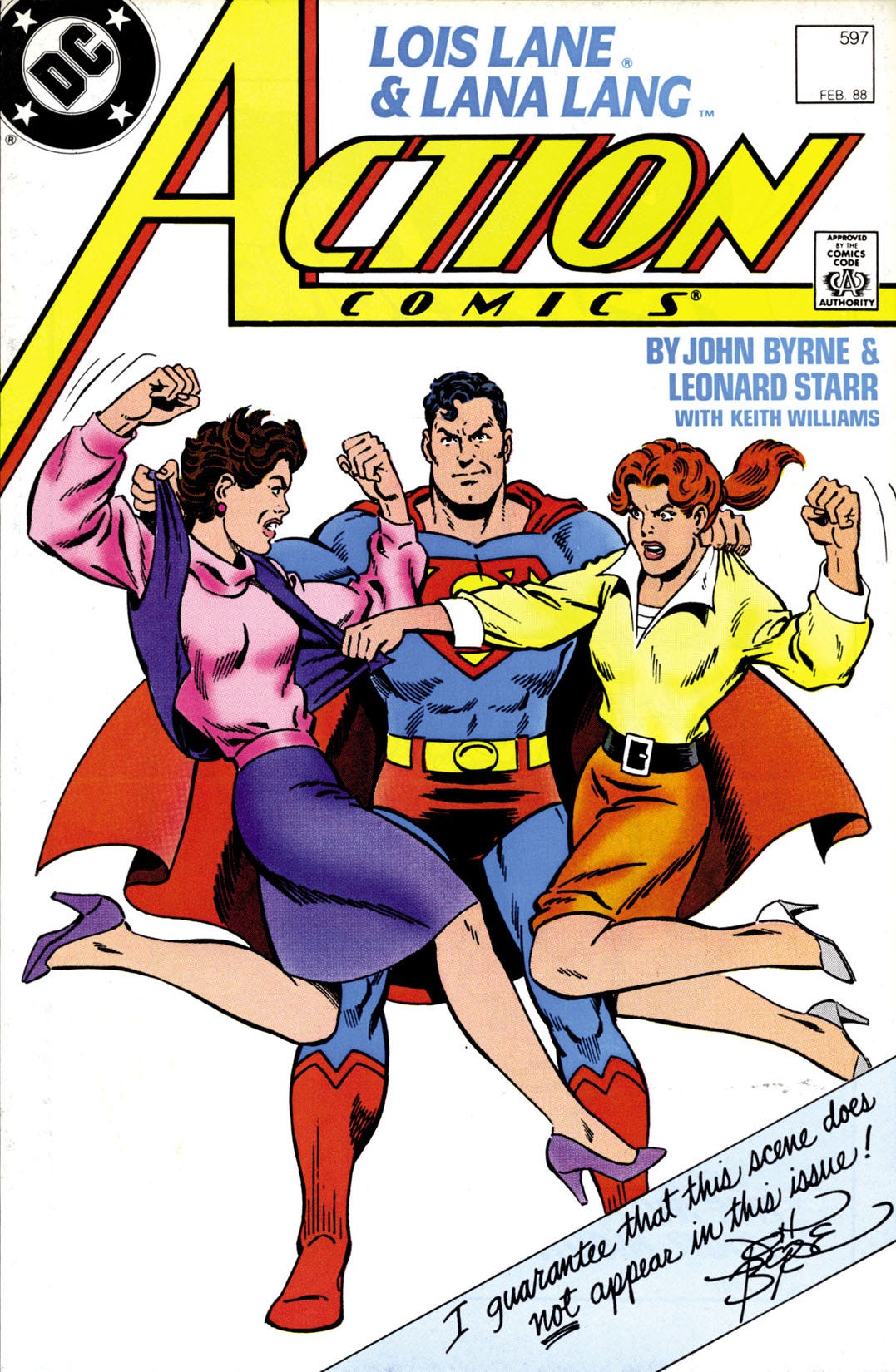This comic book cover features a vibrant and detailed illustration typical of classic superhero comics. The top of the cover prominently displays the title "Lois Lane and Lana Lang" in blue text, followed by "Action Comics" emblazoned in bold yellow letters with a red outline. In the upper left corner, a circular black-and-white stamp with four stars around it reads "DC". On the upper right, there's an empty white circle noting "February 88, 597" and "Approved by the Comics Code Authority."

In the center of the image, Superman stands tall in his iconic blue costume and red cape, with his short dark hair and a determined expression. He is holding back two women who appear to be in a heated confrontation. To his left is a woman with red hair, wearing a yellow blouse, an orange skirt, a black belt, and white high heels. To his right is another woman, depicted with brown hair, dressed in a pink shirt with a purple vest, a matching purple skirt, and purple high heels. Both women have their fists up, clearly angry, as Superman separates them with a smirk that suggests he’s experienced in handling such disputes.

Below the image, the cover credits the creators with "By John Byrne and Leonard Starr with Keith Williams" in blue letters. In the bottom right corner, a white banner humorously states, "I guarantee that this scene does not appear in this issue," followed by a signature in cursive handwriting, adding a playful touch to the cover's presentation.